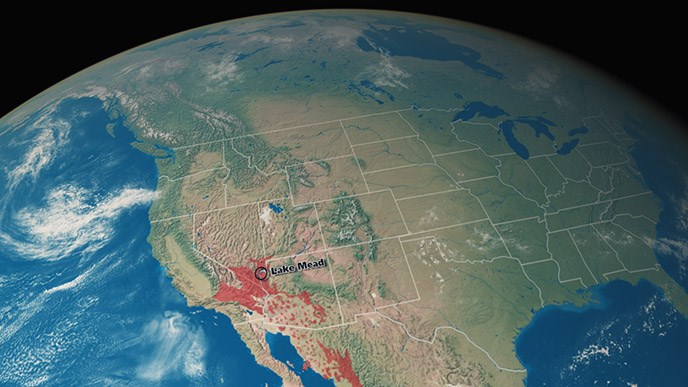This detailed render of the Earth from space focuses on North America, particularly the United States, with all state borders clearly outlined. The United States is displayed prominently in a highly recognizable map format, with a circle highlighting Lake Mead in the bottom left-hand corner. This area is annotated with a red label identifying Lake Mead. The remaining part of the United States is uniformly green. Surrounding this terrestrial depiction, the oceans are shown in blue with some white shading, indicative of the water bodies. Above, cloud formations are present but sparse over the U.S., providing a clear and unobstructed view of the land. The upper part of the continent also reveals parts of Canada, including the Great Lakes—Lake Ontario and Lake Erie—and extends down to Mexico, with notable red shaded mountains on the west coast near the border. The background is a stark black, emphasizing the spherical and somewhat rounded perspective of the Earth from space.